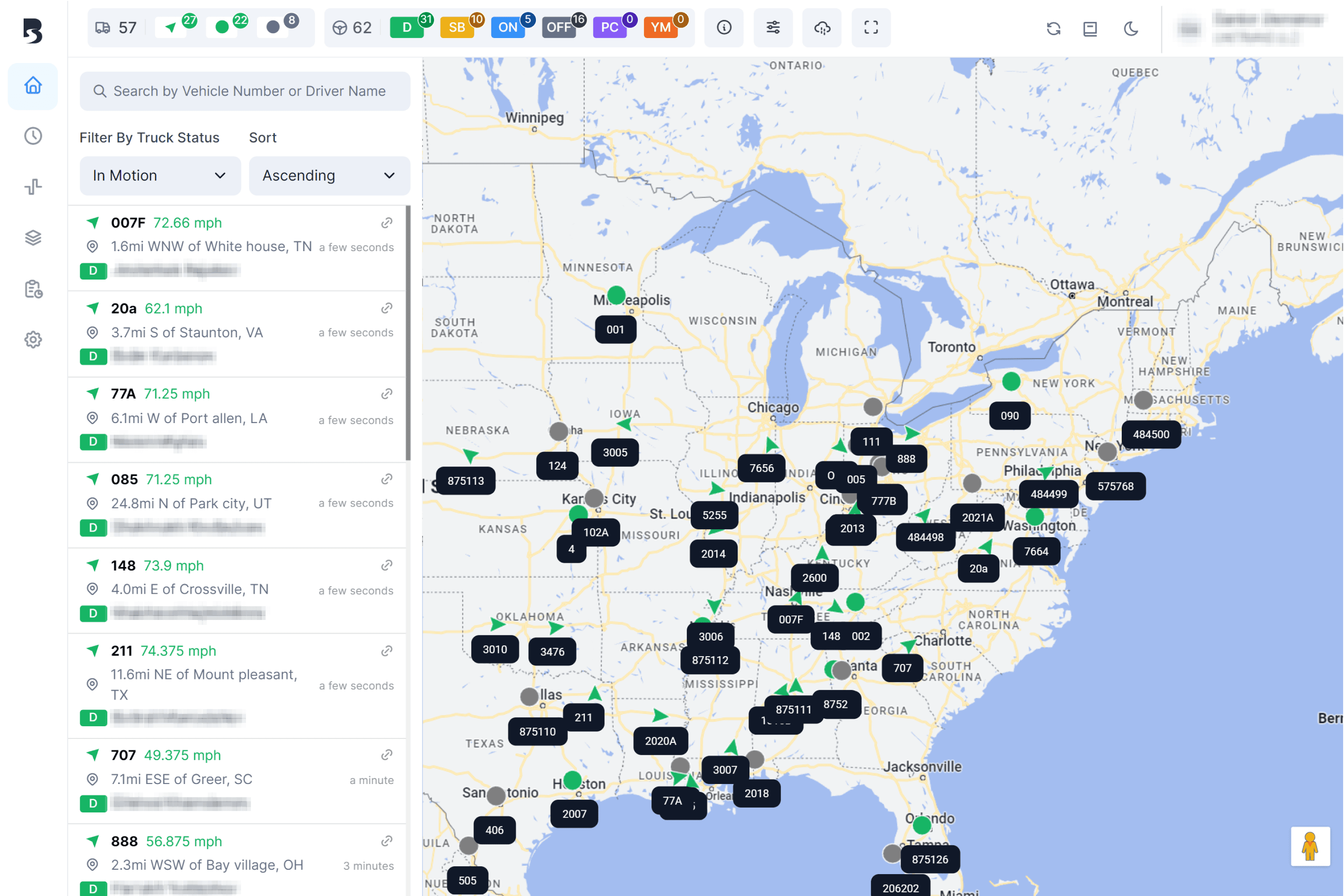The horizontally rectangular image depicts a detailed map covering the region from North Dakota to Texas, extending across the entire eastern United States. The map features a series of marked points, each enclosed in black-backgrounded boxes carrying various numerical data. On the left side of the image, there is a vertically-oriented information panel. Although much of the content in this panel is blurred, the top portion is clear, displaying options to search by vehicle number or driver name, filter by truck status (with the “in motion” status selected), and sort data in ascending order. The vertical listing pinpoints different trucks, providing specific details such as their speed and current locations.